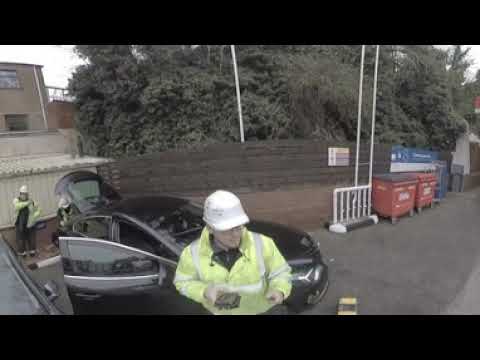The image showcases a busy construction site set in a spacious, paved area that resembles an alleyway or parking lot. Central in the frame is a worker wearing a high-visibility neon yellow jacket and a white hard hat, standing next to a small black sedan with its doors and trunk open. To the left, behind the car, two additional workers dressed in similar high-visibility clothing and hard hats are engaged in retrieving supplies from the open hatchback. Dominating the right side of the frame are two large red dumpsters positioned on the pavement, while a wooden fence runs horizontally behind the scene, partially obscuring a view of tall, overgrown trees and foliage. Beyond this, a building is vaguely visible. The area is notably clean and spacious, allowing ample room for vehicles and maneuvering.